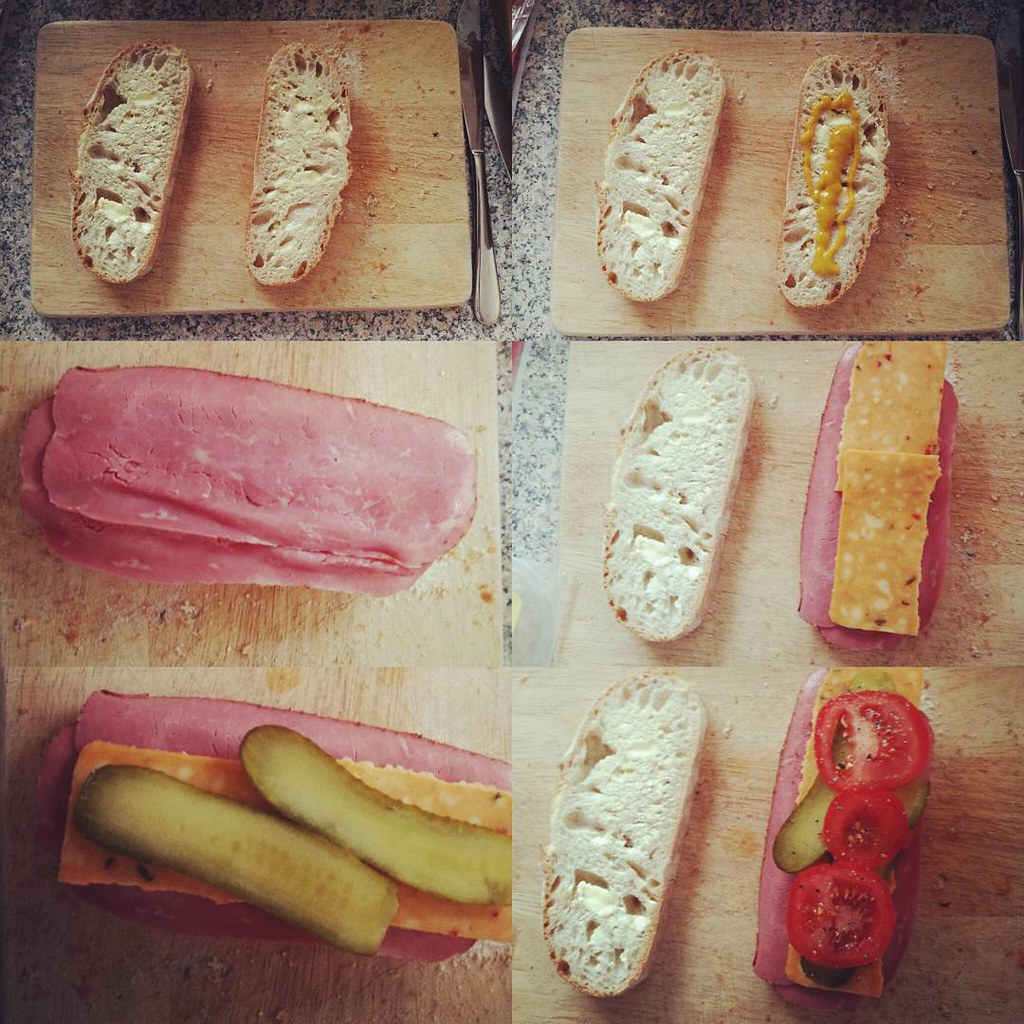A sequence of six photographs details the step-by-step assembly of a ham sandwich on a brown cutting board against a grey slab background. The first image in the top left captures two slices of bread. In the next frame, a yellow-like mustard sauce is applied to the slices. Moving to the third image, a layer of pink ham is added to one of the bread slices. The fourth image reveals slices of orange-colored cheese placed atop the ham. The fifth frame shows an additional ingredient, with two slices of pickles placed on the cheese. Finally, the last frame completes the sandwich with three tomato slices and a sprinkle of what appears to be black pepper added on top.